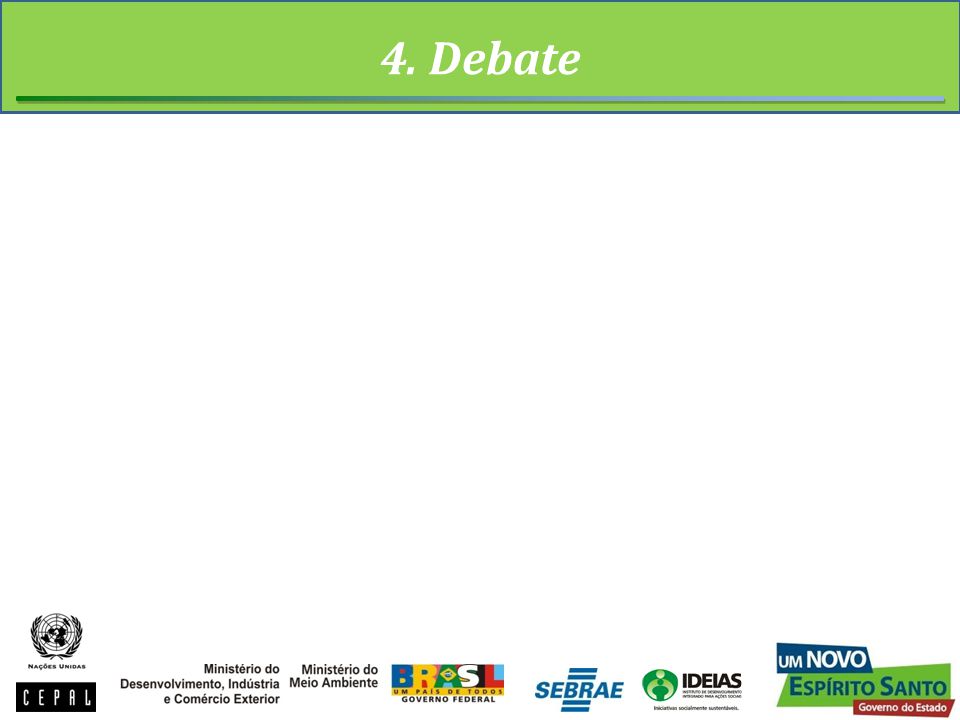The image appears to be a PowerPoint slide featuring a prominent lime green stripe across the top, bordered at the bottom by a transitioning blue line. Inside this stripe, the text "4. Debate" is prominently displayed in white, italicized font with a capital "D." Below this heading is a large expanse of white space that dominates the middle section of the slide, suggesting that something might be missing or intended to be inserted there. At the bottom of the slide, there are several logos arranged in a row, totaling about seven. These logos and accompanying text are in Portuguese, featuring the following entities: Nasa's Unidas with a globe icon; Sapon in a black rectangle; Ministerio do Desenvolvimento, Industria e Comercio Exterior; Ministerio do Mio Ambiente; Brazil, with each letter of "Brazil" in different colors; Sabrai in italics flanked by blue lines; Ideas with green icons of people; and Un Novo Espirito Santo Governo do Estado with colorful quadrilateral shapes.